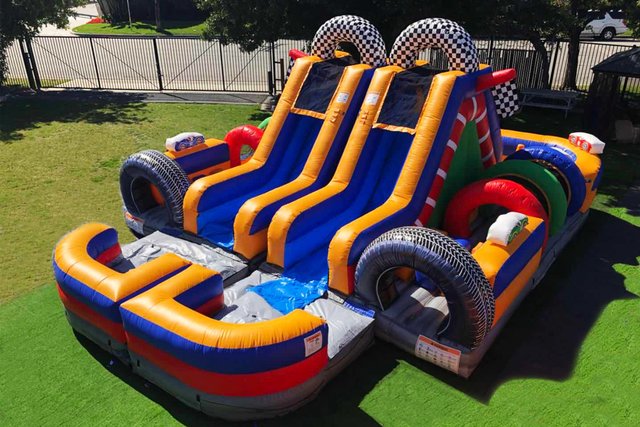The image depicts an outdoor scene, possibly a backyard or a city park, during the daytime. The focus of the photograph is an inflated children's play structure, resembling a combination of a water slide and bounce house. This inflatable structure is prominently positioned on a well-maintained green lawn, flanked by inflatable black tires on either side. The play area features two parallel slides, one yellow and one blue with yellow borders, leading down to a gray landing area. Red and green rings are positioned near the slides, adding to the vibrant play setup. 

In the background, a street can be seen beyond a large metal gate or fence, with some trees providing shade to the top right corner of the image. Despite the lively appearance of the play structure, the scene is devoid of people. The bounce house itself is colorful, incorporating shades of red, gray, blue, yellow, green, and white. The structure appears to have racing elements, with hoops at the entrance and sections designed for climbing and sliding, suggesting a playful, competitive environment. The overall setting gives an impression of a serene neighborhood space designated for children's recreation.